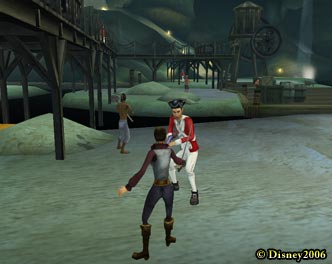This image appears to be a screenshot from an early 3D video game, reminiscent of the GameCube era. The graphics showcase the characteristic blocky textures and vibrant colors typical of that time. At the forefront, there is a pirate character dressed in a brown shirt with frilly sleeves and a flared-out collar, which is partially covered by a gray vest. The pirate is wielding a rapier or saber, engaging in combat with a British Redcoat soldier. The intense duel is set against a backdrop that hints at a nautical or coastal environment, capturing the adventurous spirit of the game.